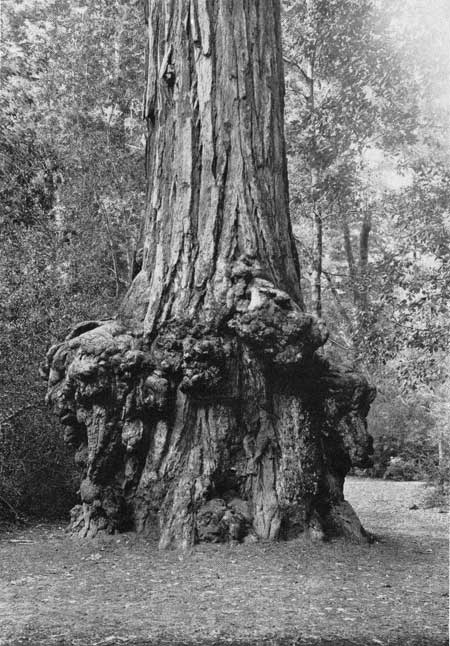This vertically aligned, black-and-white photograph features a remarkably intriguing and sizable tree trunk positioned centrally in the frame. The scene includes a foreground of short grass with scattered leaves, all depicted in various shades of gray due to the monochromatic nature of the image. The tree trunk itself is notably wide and dominates the picture, appearing to rise quite high, extending well beyond the frame. The bottom portion of the trunk is particularly fascinating; it is unusually flared and adorned with multiple growths that give it a bulky, almost cancerous appearance, distinguishing it from a typical cylindrical trunk. Above this flared base, the trunk narrows and continues upward. The surrounding area is densely wooded with tall trees flanking both sides, their thin, leafy branches contributing to a rich background. Sunlight filters through, casting a soft glow on the forest floor. The overall scene suggests an ancient, possibly centuries-old tree, standing solid and majestic amidst a tranquil, leafy forest setting.